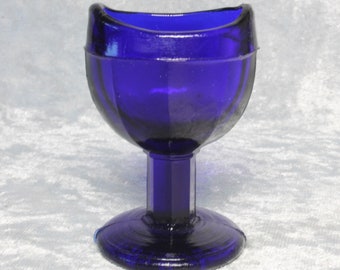This is a detailed photographic image of a glass goblet or cup, delicately captured indoors. The central object is a vivid purple glass goblet, prominently displayed on a gray marble countertop, which enhances the elegance of the setting. The goblet has a well-defined structure featuring a wide circular base that seamlessly transitions into a sturdy stem, approximately two inches tall, leading up to a broad U-shaped cup. 

The cup appears to have a dual-layer design— an outer layer of lighter purple glass fused over a darker purple inner layer, adding both depth and richness to the visual. The outer and inner layers form a thicker composite that accentuates the goblet's robust yet refined aesthetic. The cup's wide brim slightly undulates, and there's an impression of melted wax around the edges, suggesting it could also function as a candle holder. 

In the background, a textured mix of light gray and white hues evokes the serene feel of flowing water. This textured backdrop, combined with the glass reflections and subtle flashes captured in the photo, contributes to the overall serene and elegant ambiance of the image. There is no text present, allowing the clear and detailed design of the goblet to remain the focal point.